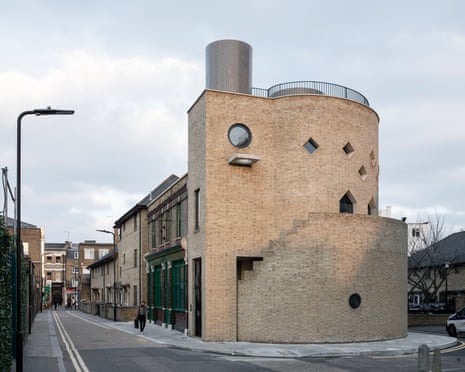The image captures a gloomy winter midday scene of a distinctive city block lined with two-story light-colored brick buildings. The focal point is a peculiar, narrow building with a rounded shape designed to fit the curved street and sidewalk alignment. The building has unique diamond-shaped and circular windows and is topped with a metal deck and fencing, possibly for observational use, and a cylindrical structure likely holding equipment or water. The only tree visible is leafless, confirming the season. A single person walks up the left side of the relatively quiet sidewalk. The combination of overcast skies and the lone pedestrian highlights the stillness of this part of town.